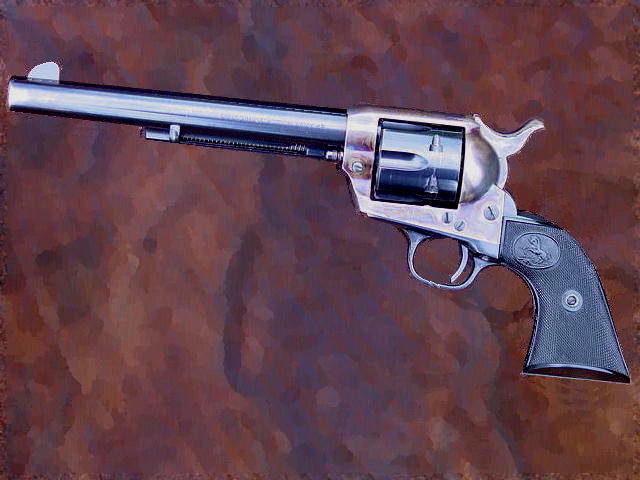The image depicts a shiny, relatively new revolver with a distinct silver finish. The gun, appearing old-fashioned in its design, is positioned with the handle on the right and the barrel on the left. The long barrel, silver with a hint of a blue sheen, extends prominently. The black handle features a small circular logo resembling a horse and is secured by three visible screws. The cylinder, designed for five shots, is also silver. The blurred background consists of various shades of brown, rust, tan, and hints of purple, giving an almost spotted, textured appearance that contrasts with the sharp focus on the revolver.